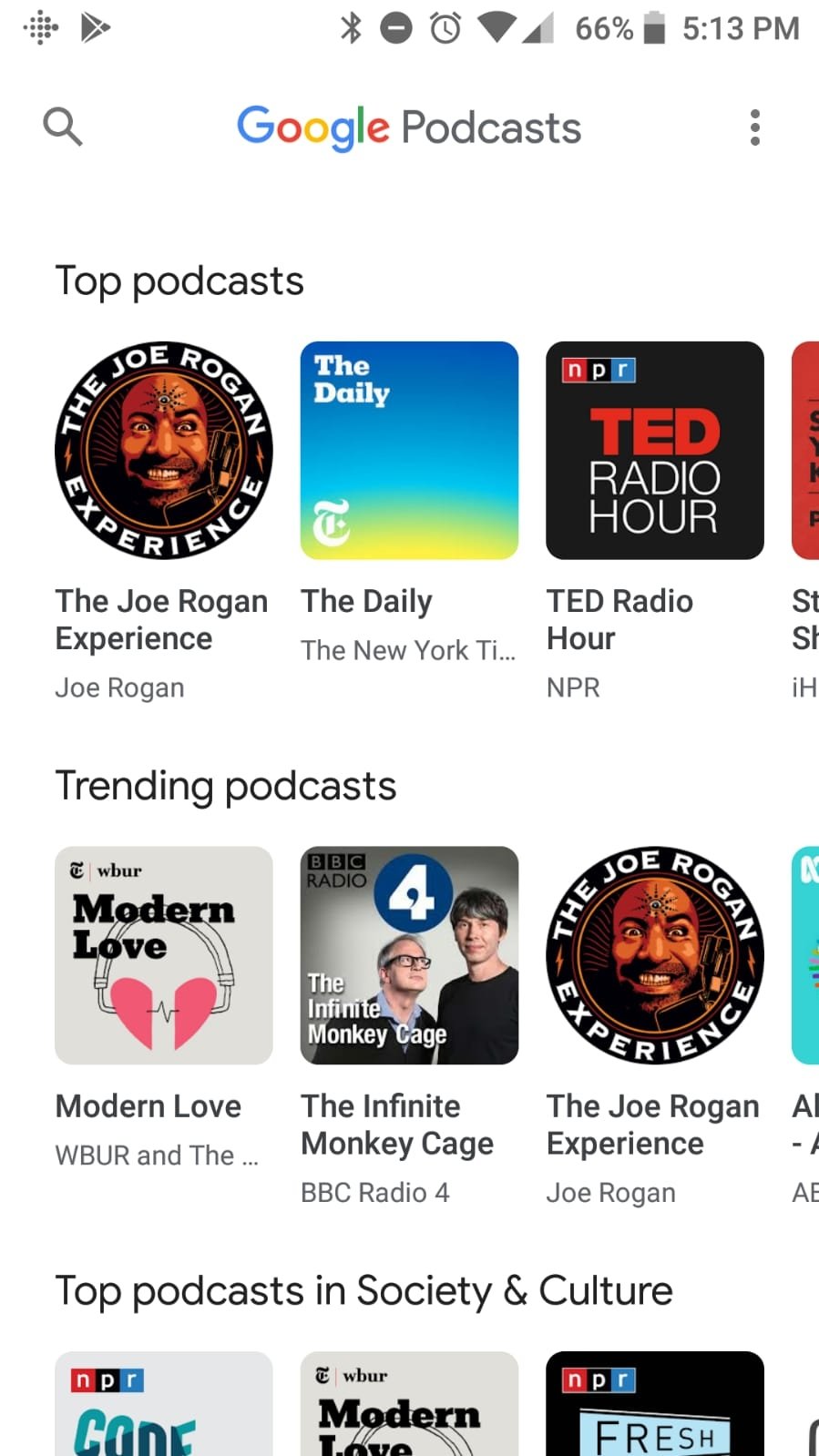This is a detailed screenshot of a smartphone displaying the Google Podcasts app. The phone's battery is at 66%, the time is 5:13 p.m., and the signal strength is weak. The interface of the app has a white background. 

At the top, the app identifies itself with "Google Podcasts." Below, it lists the top podcasts, starting with "The Joe Rogan Experience," followed by "The Daily" from The New York Times, and "TED Radio Hour" by NPR.

Further down, the app highlights trending podcasts, including "Modern Love" from WBUR, which is visually depicted using an image of a pair of headphones with each ear pad forming one-half of a heart. Following this is "The Infinite Monkey Cage," a BBC Radio 4 podcast featuring an image of two men standing. The list also includes "The Joe Rogan Experience" again among the trending titles, while some other trending podcasts are cut off and not fully visible in the screenshot.